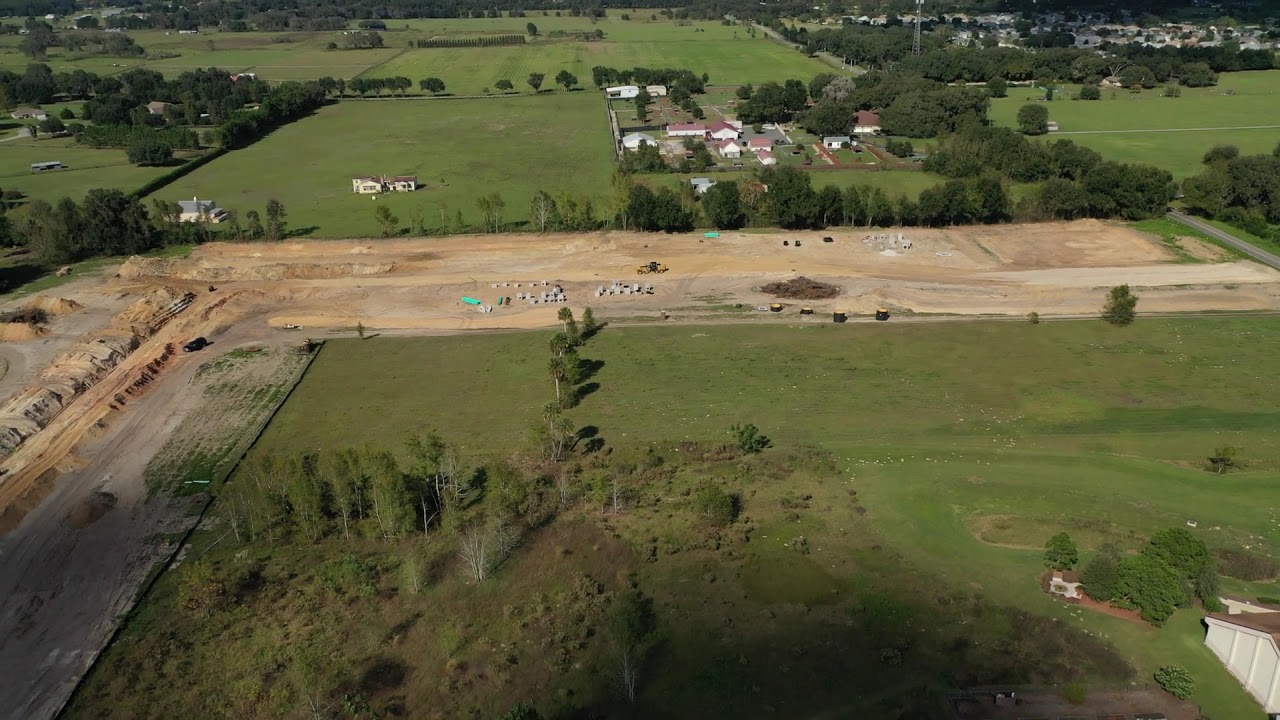The image offers an extensive aerial view of a sprawling rural region, teeming with fields, roads, and scattered houses. In the immediate foreground, numerous grassy fields are laid out in a grid-like pattern, dotted with clusters of trees. Among these fields, one can discern areas designated for farming, likely fenced off and perhaps containing livestock such as sheep. Adjacent to these fields lies a section of freshly graded dirt, suggesting an active construction site with trailers and a road being cut out by a tractor, possibly for a forthcoming residential project.

As the eye moves further into the distance, the terrain shifts to muddy topsoil areas, which blend into more farmland stretching out across the landscape. These farms are interspersed with rectangular plots and small clusters of houses, predominantly on the right-hand side, with a few isolated homes on the left. Further out, towards the top-right of the image, the density of houses increases, hinting at a suburban fringe of a nearby town or city, characterized by more concentrated tree cover and residential properties. A long, two-lane asphalt road weaves its way through this picturesque yet industrious countryside, tying the various elements of this diverse environment together.